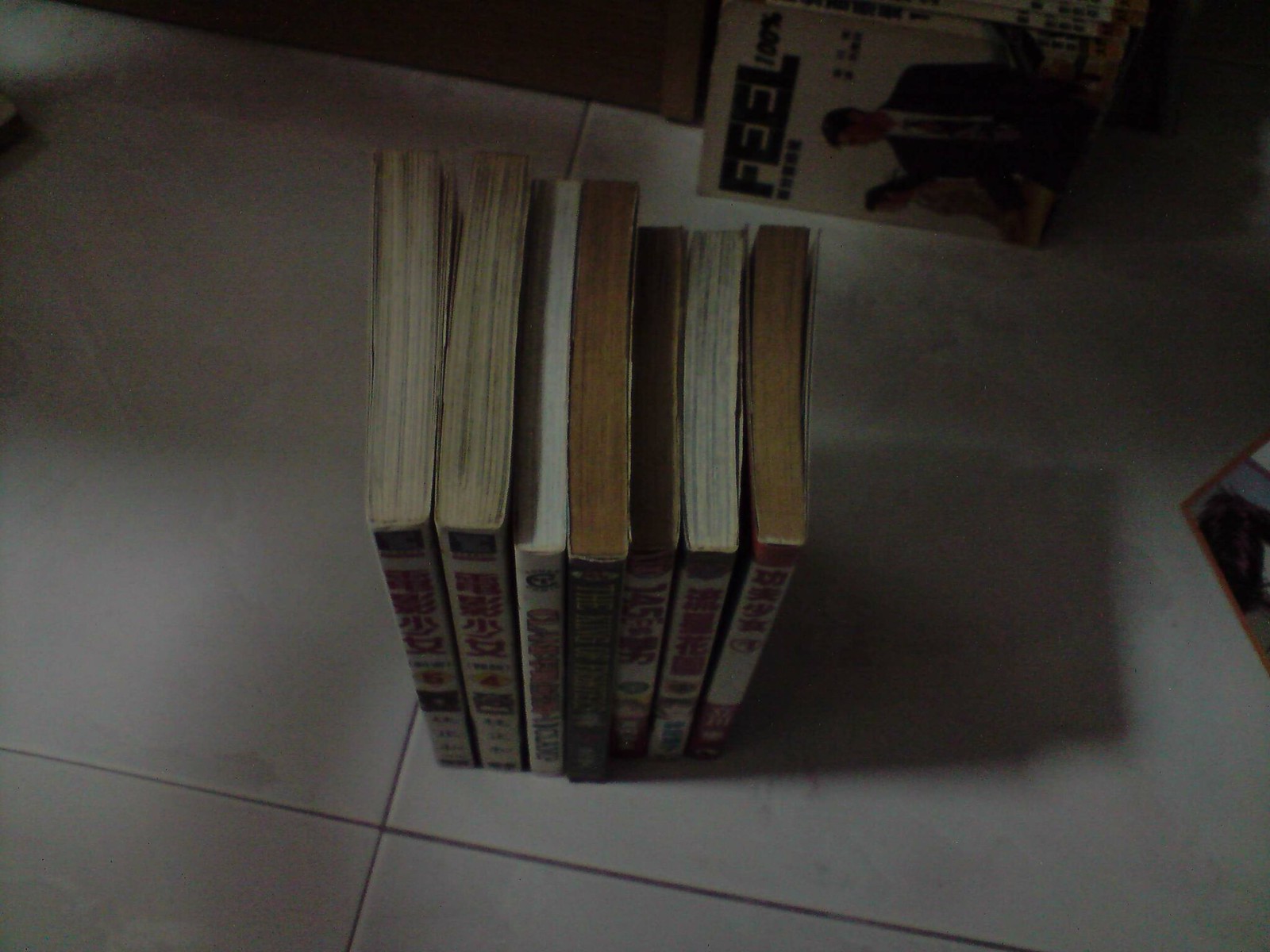This photograph captures an overhead view of seven vertically positioned books standing on a white tile floor with large square tiles. The room is extremely dark, casting distinct shadows of the books onto the floor. The spines of the books face forward, though the lettering is largely illegible, with some Chinese writing visible on a few. Notably, two books on the left appear white with red writing and black stickers, while the central book is black with yellow accents. To the right, a lone book labeled "Feel" lies horizontally, depicting a man in a suit and tie on its cover, alongside what appears to be a woman to his left. The overall scene is barely illuminated, emphasizing the shadowy and muted ambiance of the setting.